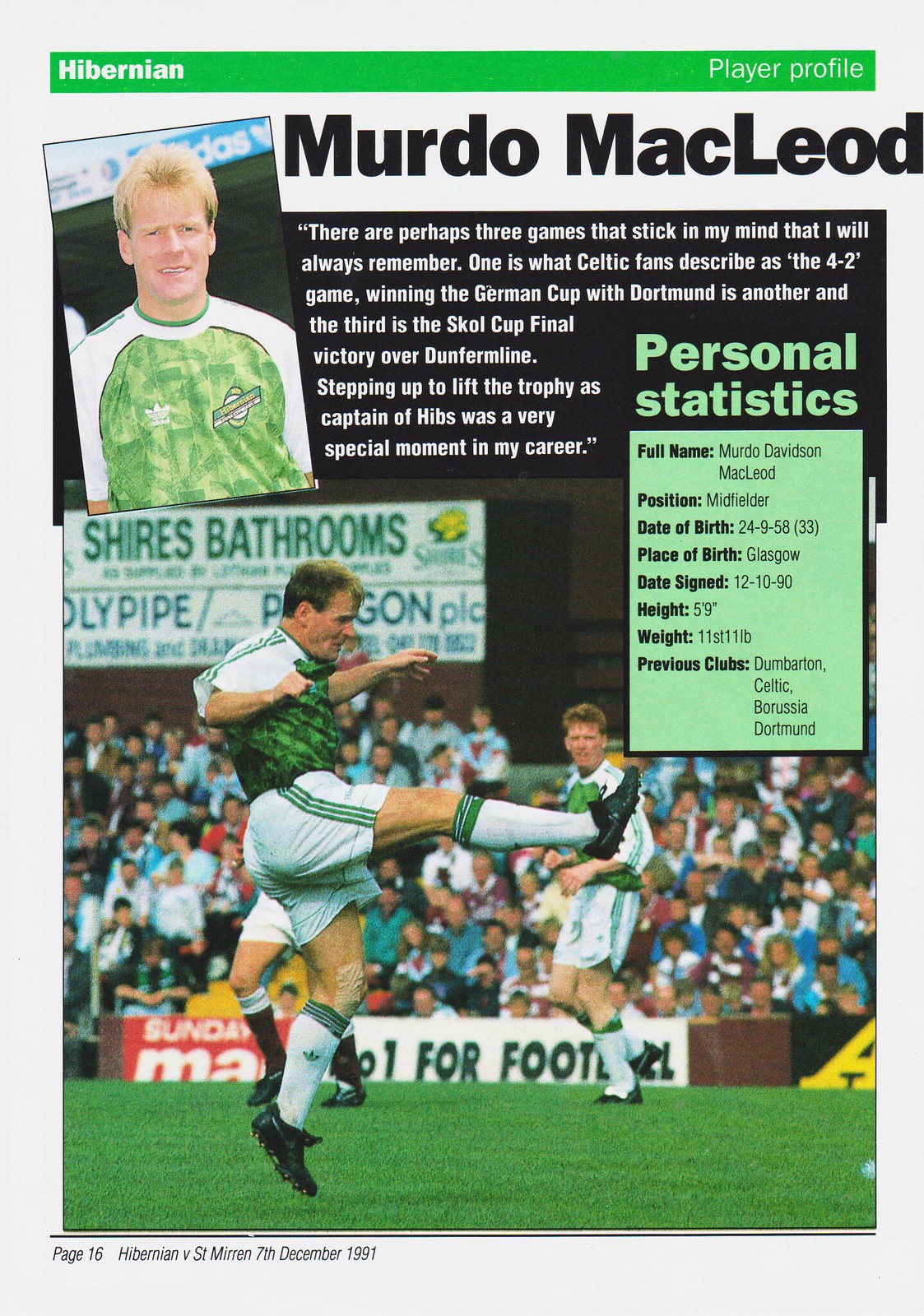The magazine page, dated December 7, 1991, from an unspecified publication, features a detailed profile of Hibernian soccer player Murdo McLeod. The page is in full color, with a green bar across the top that reads "Hibernian" on the left and "Player Profile" on the right. Below, Murdo McLeod’s name is highlighted in bold black font. 

A portrait of McLeod, a blond man with short-cropped hair and light skin, is inset on the left, showing him wearing a green soccer jersey with white sleeves. A biography of McLeod appears alongside the photo, though the font is too small to read in detail. The text includes memorable quotes from McLeod about significant games in his career, such as winning the German Cup with Dortmund and lifting the Skol Cup as captain of Hibs.

To the right of the biography is a green box containing his personal statistics, though these details are also too small to discern. Below this, a dynamic, full-color action shot captures McLeod on the soccer field mid-kick, donning Hibernian's green and white kit: white shorts with green stripes, white socks with green bands at the top, and black shoes. In the background, another teammate is visible, along with a packed stadium and an advertisement for the Sunday Mail. The page number "16" is in the bottom right corner, denoting this magazine excerpt focuses on Hibernian versus St. Mirren.